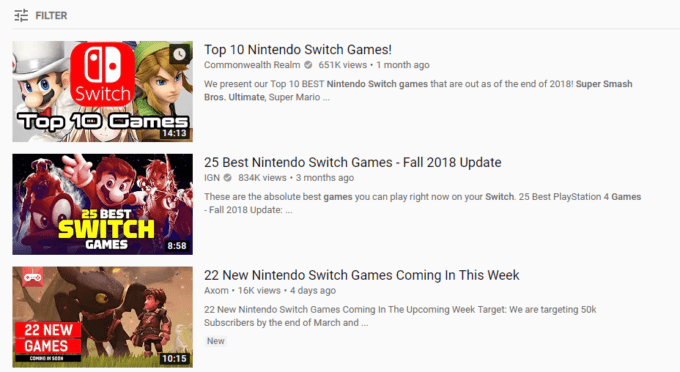The image showcases a YouTube search results page with a light gray background. The top left corner features a "Filter" icon for refining the search results. Three videos are displayed on the screen, each related to Nintendo Switch games.

1. **First Video:**
   - **Title:** Top 10 Nintendo Switch Games
   - **Channel:** Commonwealth Unreal
   - **Views:** 651k
   - **Date:** Uploaded one month ago
   - **Duration:** 14 minutes and 13 seconds
   - **Description:** "We present our top 10 best Nintendo Switch games that are out as of the end of 2018, including Super Smash Bros Ultimate and Super Mario."
   - **Thumbnail:** Features a red and white Nintendo Switch controller with text that reads "Top 10 Games."
   
2. **Second Video:**
   - **Title:** 25 Best Nintendo Switch Games for 2018 (Update)
   - **Channel:** IGN
   - **Views:** 834k
   - **Date:** Uploaded three months ago
   - **Description:** "These are the absolute best games you can play right now on your Switch, updated for 2018."
   - **Thumbnail:** Contains text that reads "25 Best Switch Games" in white and yellow.

3. **Third Video:**
   - **Title:** 22 Nintendo Switch Games Coming This Week
   - **Channel:** Axon
   - **Views:** 16k
   - **Date:** Uploaded four days ago
   - **Description:** "22 Nintendo Switch games coming in the upcoming week. We are targeting 50k subscribers by the end of March."
   - **Thumbnail:** Features the text "22 New Games" on a red background.